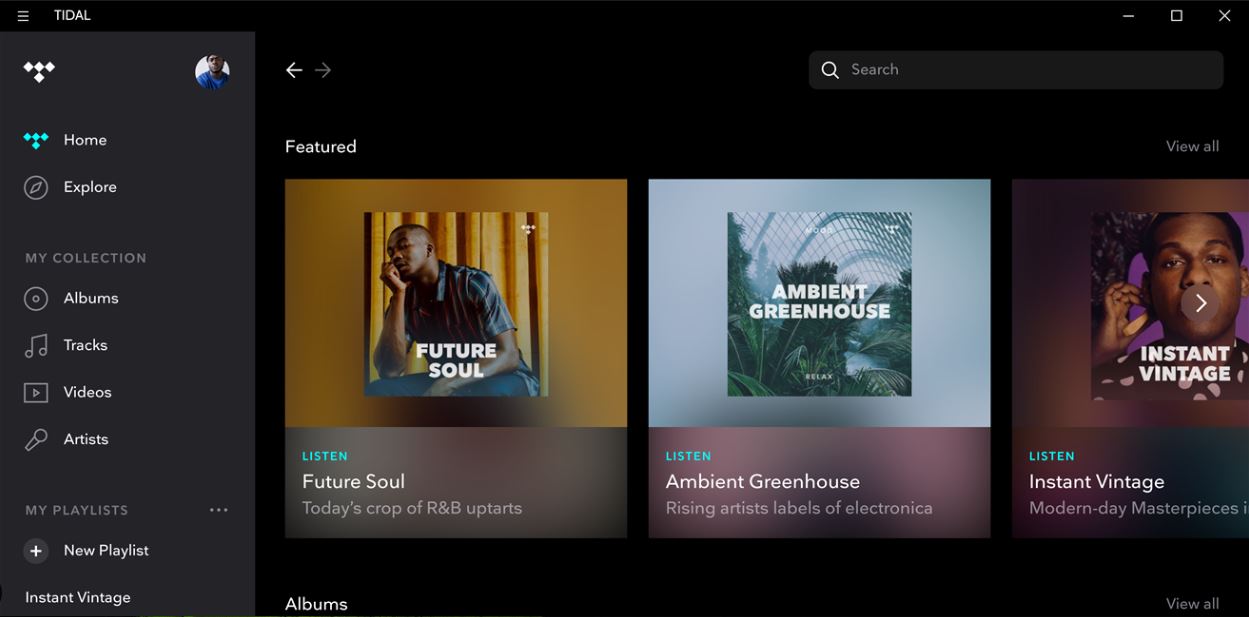This is an image capturing the homepage of a music streaming application displayed on a computer screen. The interface is split into two distinct sections: a black background on the right and a gray background on the left. At the very top, the word "Title" is prominently displayed in white.

The gray section on the left is organized into various categories. At the top, "Home" is listed, with "Explore" directly beneath it. Moving down, there's a section labeled "My Collection" with subcategories: "Albums," "Tracks," "Videos," and "Artists." Below that, a section titled "My Playlist" includes an option to add a "New Playlist." A user profile icon, depicting a male figure in a blue shirt, is situated in the upper right corner of this gray area.

The black section on the right features a search bar located at the top right. Below that, there are three highlighted segments, each appearing as album covers. The section is labeled "Featured" in the upper left corner. 

The first album cover displays a black male set against a brown background, titled "Future Soul." In white text, it states, "Listen - Future Soul: Today's crop of R&B upstarts."

The middle album cover has a gray background with an image of a greenhouse, named "Ambient Greenhouse." The descriptive text reads, "Listen - Ambient Greenhouse: Rising artists and labels of electronica."

The rightmost album cover features another black male and is titled "Instant Vintage." Its description reads, "Listen - Instant Vintage: Modern-day masterpieces."